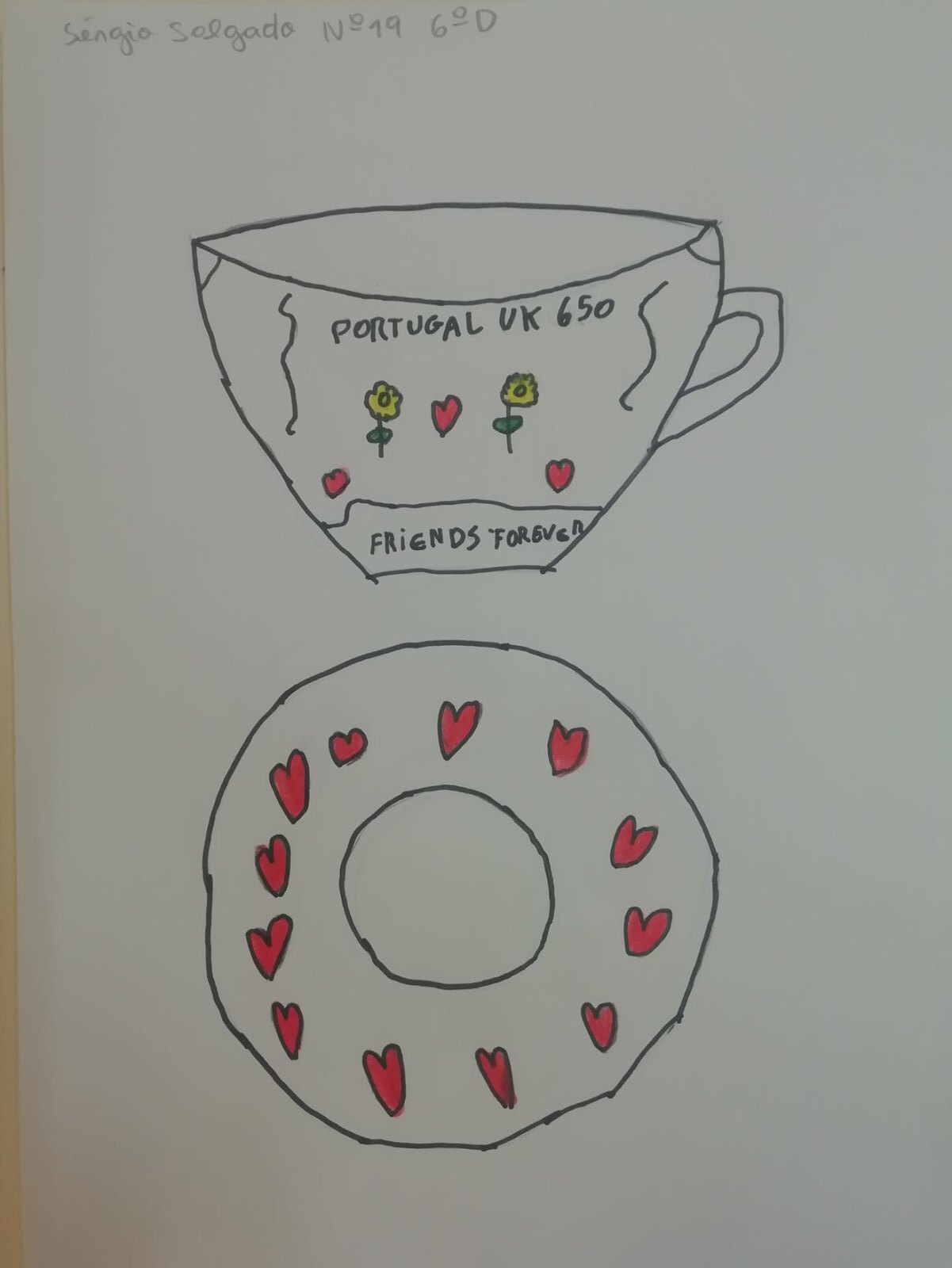This detailed description is for a photograph of a whimsical, kid-style drawing of a teacup and saucer, rendered on a white sheet of paper with a black pen or marker. The teacup, depicted with a shaky black outline, is in the front view with the handle on the right side. It prominently displays the text "Portugal UK 650" in all caps, flanked by two squiggly lines. Below this, two alternating tiers of elements consist of a series of red hearts and yellow-green flowers, specifically arranged as a red heart, flower, red heart, flower, and another red heart. Beneath these, a curved horizontal squiggly line features the inscription "Friends Forever."

The accompanying saucer is seen from a top-down perspective, though its shape, like that of the teacup, is imperfect and roughly circular. Around its perimeter, it bears twelve freehand red hearts of varying sizes and shapes, with another smaller circle indicating the center indentation for the teacup. Additionally, at the top left of the drawing, inscriptions include "Sergio Salgada," "N19," and "6D." The artistry is enhanced with bright spots of color: the hearts are vivid red while the flowers are highlighted in yellow with green leaves. The overall presentation is playful and vibrant, capturing a childlike charm.